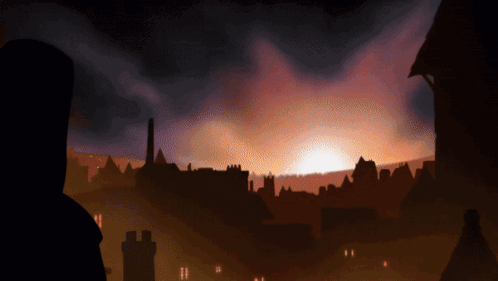This small, horizontal, rectangular image appears to capture either a sunrise or a sunset, shrouded mostly in darkness. The top and sides are enveloped in irregularly shaped, billowing dark clouds, with hints of a reddish hue, possibly signifying trees or additional clouds. A bright orange-brown glow illuminates the horizon, where the sun is either ascending or descending, creating an eerie contrast against the murky sky.

In the foreground, obscured in the dim light, are indistinct shapes that could be either a grassy area or a collection of buildings and trees. Notably, there appear to be outlines of structures with pointed and jagged edges, reminiscent of a village set in a sandy, desert-like terrain, perhaps evoking images of an Arabic village. Scattered specks of light suggest reflections from windows or small light sources.

Additionally, near the bottom left, faint images of two figures may be discerned standing and gazing at the view, enhancing the scene's mysterious and contemplative atmosphere.